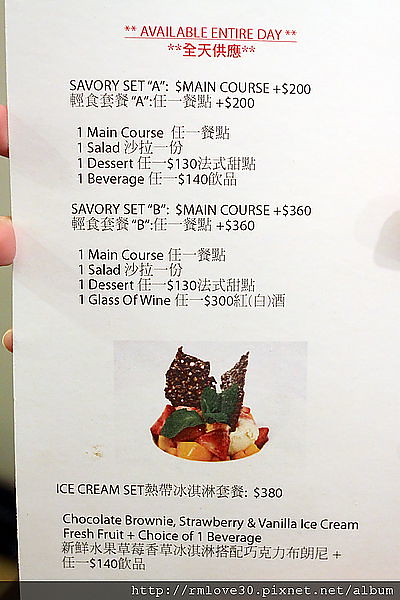The photograph shows a hand holding a paper menu, with three fingers visible on the left side. The menu features both English and Chinese text, printed in black on a white background. At the top, in red font with asterisks, it reads "Available Entire Day." Below this, Chinese characters accompany the English descriptions and prices.

The first section lists "Savory Set A," detailing "1 Main Course, 1 Salad, 1 Dessert, 1 Beverage," priced at $200, with corresponding Chinese translations. The next section describes "Savory Set B," which includes "1 Main Course, 1 Salad, 1 Dessert, 1 Glass of Wine," priced at $360, again with Chinese translations.

A colorful image of a dessert featuring strawberries, mango, and decorative elements is displayed beneath these sets. This is labeled as "Ice Cream Set," priced at $380, and includes "Chocolate Brownie, Strawberry and Vanilla Ice Cream, Fresh Fruit, plus 1 Choice of Beverage," all accompanied by Chinese translations.

Towards the bottom of the menu, an overlay in dark gray, slightly transparent, contains the text "http://rmlove30.pixnet.net/album," indicating a digital addition to the image.